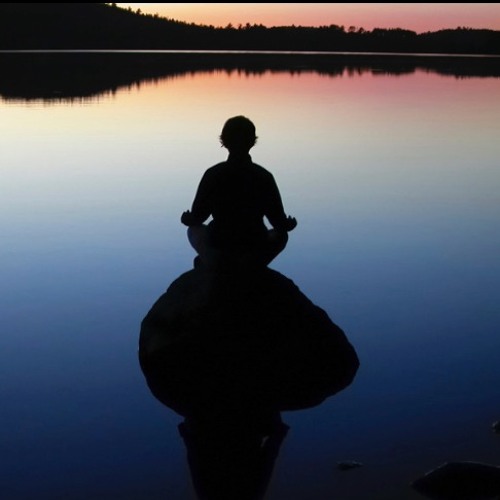In this stunning, serene photograph of a calm lake, a person—possibly a young woman—sits cross-legged on a large rock that emerges from the water. The rock and figure are silhouetted against the radiant colors of a sunset, with the western sky glowing in rich hues of red, pink, and yellow that seamlessly blend into the reflective surface of the still water below. Surrounding the lake are darkened trees, adding to the tranquil atmosphere. The person appears to be meditating, with arms resting on their knees, seemingly absorbed in the peaceful beauty of the moment. The overall scene exudes a sense of calm and introspection, enhanced by the mirror-like quality of the water reflecting the vivid, serene sunset.